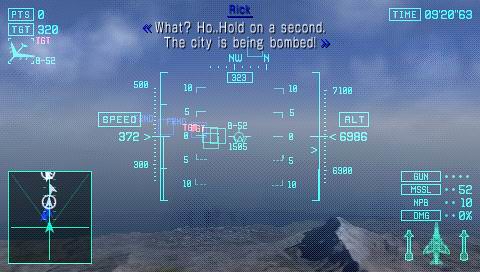This is a detailed screenshot from a fighter pilot video game. In the bottom left corner, a green-colored mini-map features arrows indicating airborne objects. The bottom right corner displays a user interface (UI) element labeled “Gun, Missile, NPD, and Damage.” The missile count reads 52, NPD at 10, and damage is 0%, accompanied by an icon of a fighter jet with two missiles on each side.

In the upper right corner, the time reads 92:06.3. The landscape below showcases a mountain range against a blue sky. Speed is indicated at 372 on a gauge ranging from 300 to 500, while altitude is shown as 6986 on a scale from 6900 to 7100. A compass pointing Northwest at 323 is also present.

At the top of the screen, the name Rick is displayed alongside a dramatic message, "Wait, hold on a second, the city is being bombed."